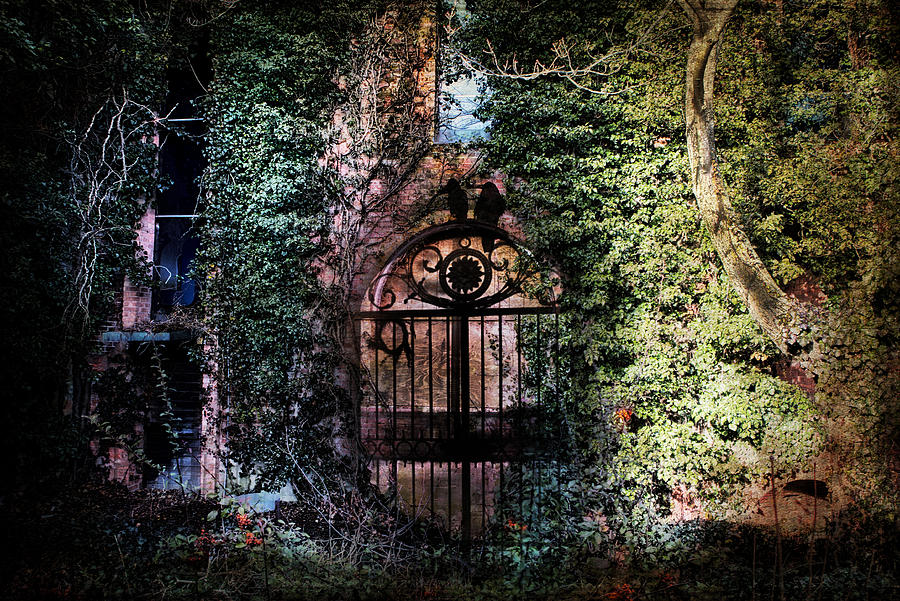In this dramatically contrasting scene, you are greeted by an ornate black iron bar gate at the center, featuring an archway embellished with intricate designs. The entire gate is enveloped in varying hues of ivy—on the left side, the ivy has a dark, forest-green coloration, while on the right, it transitions into a light, yellowish-green under the rays of the sun. The gate itself exudes an eerie, almost magical aura, enhanced by the presence of two black ravens perched atop. The gate leads to an old, weathered building with a reddish-brown facade peeking through the lush foliage, suggesting an air of deliberate neglect or vintage charm. In the background, a hint of blue sky is visible amidst the overwhelming greenery, carrying a sense of tranquility. This surreal image, possibly a digitally altered photograph or painting, plays on the stark contrast between light and dark, old and new, evoking a sense of mystery and enchantment.